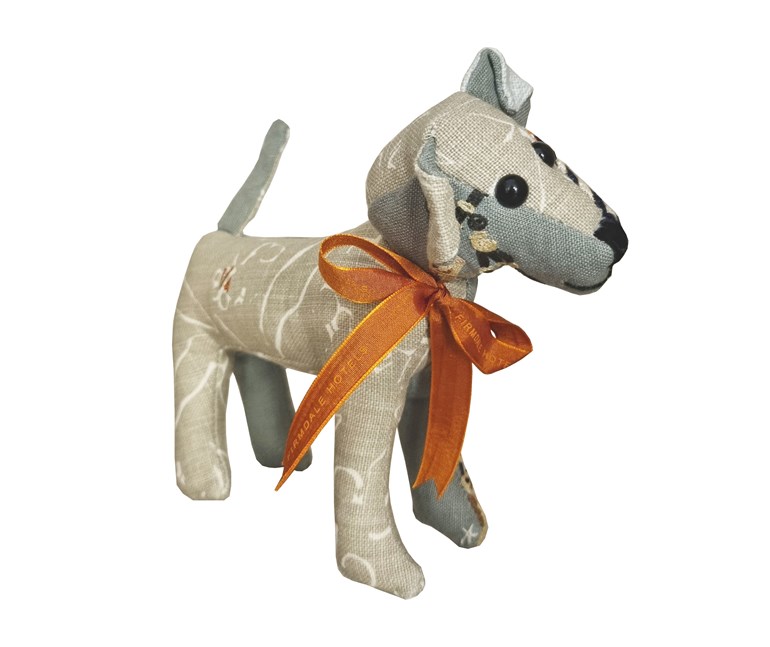This color photograph, presented in a square format, captures a handmade stuffed toy in the shape of a dog. Made from a light brown and light blue tweed-like fabric adorned with a white intermittent pattern, the dog stands on all fours with its head slightly tilted and facing to the right. Its playful expression is marked by black button eyes and a small stitched nose and mouth. The dog features curved, flopped-over ears, and a tail sticking straight up. A satin bow, rust to dark orange in color, adorned with the words "Ferndale Hotel" is tied around the dog's neck, suggesting it may be a promotional gift. The background is a pristine white, highlighting the toy's detailed craftsmanship in a style that mirrors photographic realism, indicative of product photography.